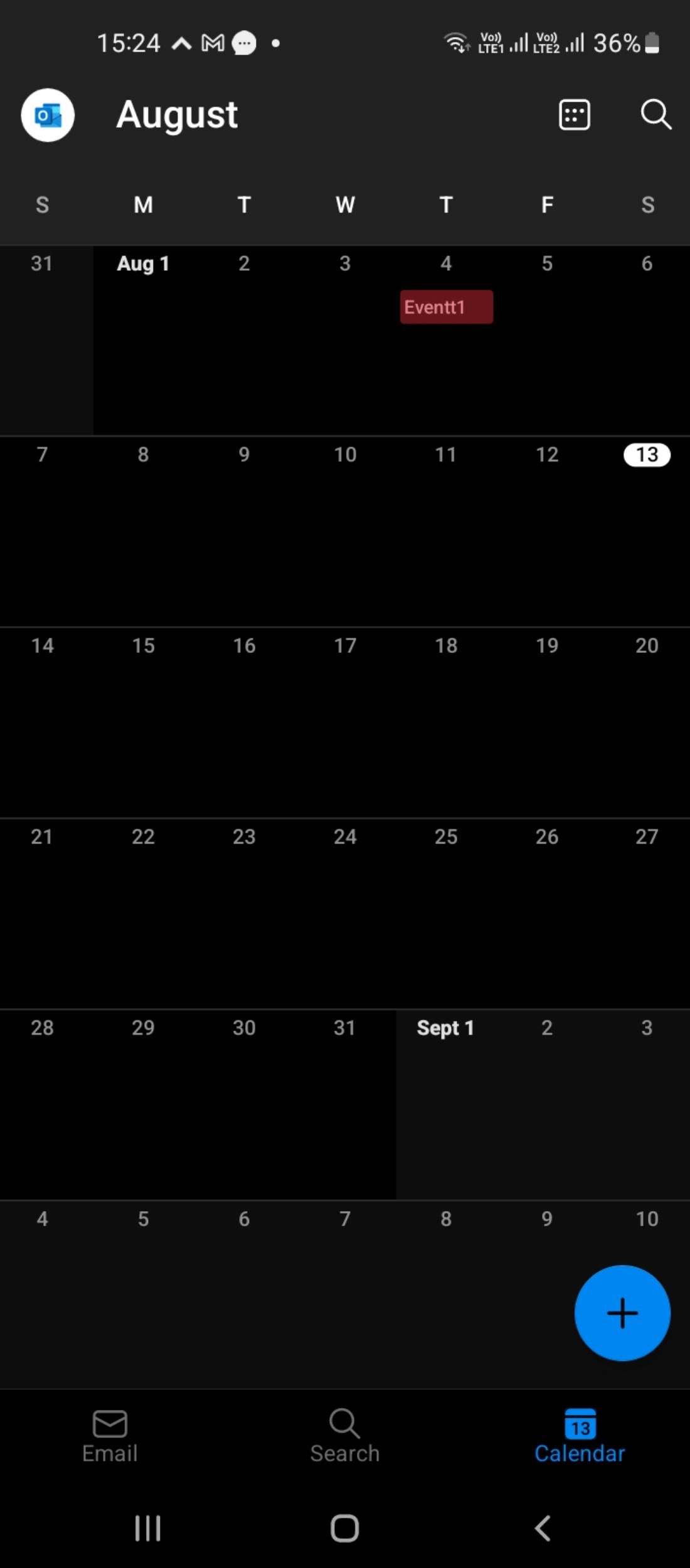The image features a black background with various UI elements arranged methodically. 

In the top-left corner, white text reads "15-24" accompanied by an arrow pointing upwards. To the top-right, it indicates a battery life of 36%, suggesting it's rather low. There are also icons signifying active Wi-Fi and sound settings.

On the left side, in the middle, is a white circle containing the Microsoft Outlook logo in blue. Adjacent to it, "August" is written in white font. Beside this is a magnifying glass icon representing the search function.

Central to the image is a calendar layout. Days are represented by their initials—"SMTWTFS." Below this header, dates are arranged accordingly: July 31st (Sunday), followed by August 1st (Monday), 2nd (Tuesday), 3rd (Wednesday), and 4th (Thursday). Notably, below these dates, the text "Event One" is displayed in white font against a black-and-red background. 

Further down the calendar, the 13th is highlighted in white, designating it a Saturday. A few lines below this, September 1st (a Thursday) is also highlighted in white. 

At the very bottom right of the image, there is a blue circle with a white plus sign within it. To its left lies an email icon accompanied by the words "Email Search Calendar." The 13th is highlighted in a blue box, and three vertical lines appear just left of center.

The central square contains a left arrow, denoting a navigational option within the calendar interface.